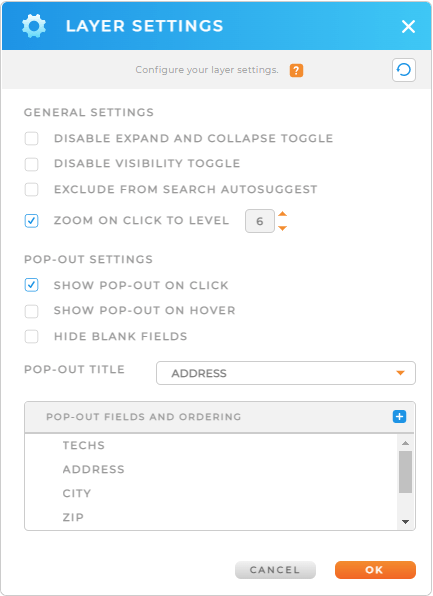This is a detailed smartphone screenshot of a "Settings" page, characterized by a gradient banner that transitions from blue to baby blue towards the right, where a close-out "X" icon is located. On the left side of the banner, a settings wheel icon signifies the settings menu.

The main settings panel is light gray, featuring text in a lighter gray that reads "Configure Your Layout Settings" accompanied by a question mark in an orange square, suggesting a help tooltip. To the right of this text is a refresh button.

The first section under this panel is labeled "General Settings", containing multiple checkboxes arranged vertically. These options include:
1. "Disable Expand and Collapse Toggle"
2. "Disable Visibility Toggle"
3. "Exclude from Search Auto Search Suggest"
4. "Zoom on Click to Level" — the only checkbox that is checked.

Adjacent to this section is a numeric input box displaying the number '6'. This box includes up and down arrows for incrementing or decrementing the value.

The next section is titled "Pop Out Settings", which includes the following checkboxes:
1. "Show Pop Out on Click" — this box is checked.
2. "Show Pop Out on Hover"
3. "Hide Blank Fields"

Below these options, there's a field labeled "Pop Out Title" followed by a text box for entering an address, which has a dropdown arrow for additional selections.

The final section titled "Pop Out Fields and Ordering" features a plus icon to the right and contains the following text fields within a box: Address, City, Zip Code. At the bottom right of the panel, there are two buttons labeled "Cancel" and "Okay", providing options to either discard or save the settings changes.